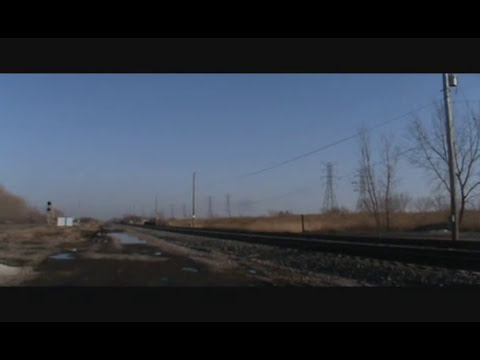The image depicts a rural, wintry landscape featuring a set of railroad tracks extending into the horizon under a clear blue sky. The foreground shows the dark brown tracks laid upon a gravel bed, devoid of any trains. To the right of the tracks lies a barren field interspersed with spindly, leafless trees, suggestive of the winter season. Alongside the tracks run several thin utility poles connected by taut wires, potentially for electricity or communication, with taller power towers visible in the distant background. On the left side of the tracks, the landscape consists of dry brown vegetation, resembling twigs or brush. The scene also includes a light warning signal and an indistinct sign on the left side. Framed by cinematic black and dark gray bars at the top and bottom, the image exudes a desolate yet structured aesthetic, emphasizing both natural and man-made elements without any human presence.